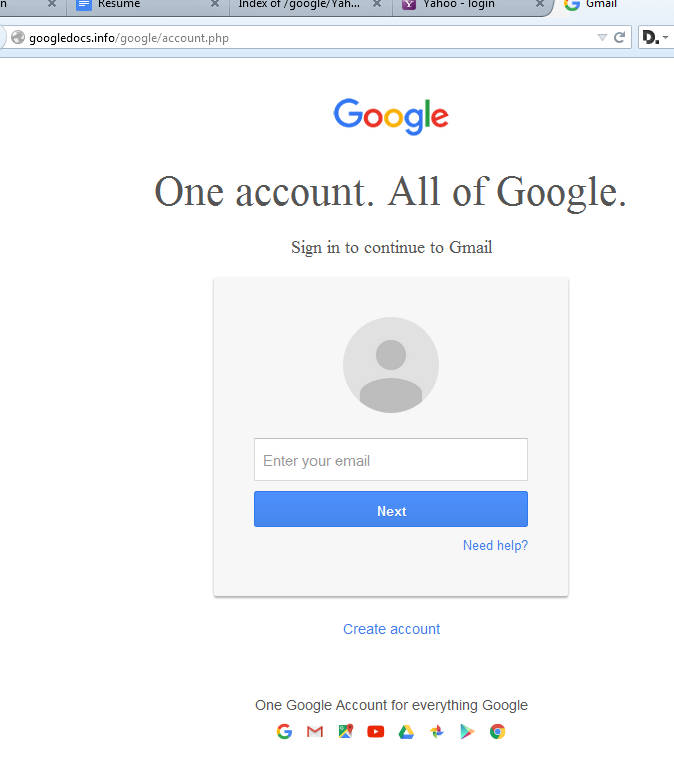The image depicts a computer screen displaying a webpage in a web browser, with multiple browser tabs visible at the top. Specifically, the browser is open to a Gmail sign-in page. The visible tabs include at least five, but there may be more since the image is cropped and zoomed in to focus on one section of the screen. The highlighted tab reads "Gmail," indicating the active page.

The URL displayed in the address bar is "Google Docs dot info slash Google slash account dot PHP." Below that, the Google logo is prominently visible, displaying the company's iconic multicolored lettering in blue, red, yellow, and green.

The page headline reads in bold black text, "One account. All of Google." Below this, smaller black text instructs the user to "Sign in to continue to Gmail."

Centered on the page is a grey box featuring a circular icon with a dark grey silhouette of a person, symbolizing a user profile. Directly below this icon, a rectangular field prompts the user to "Enter your email" in grey text. A blue "Next" button is situated beneath this field, its text in white. Additional blue text options include "Need help?" and "Create account."